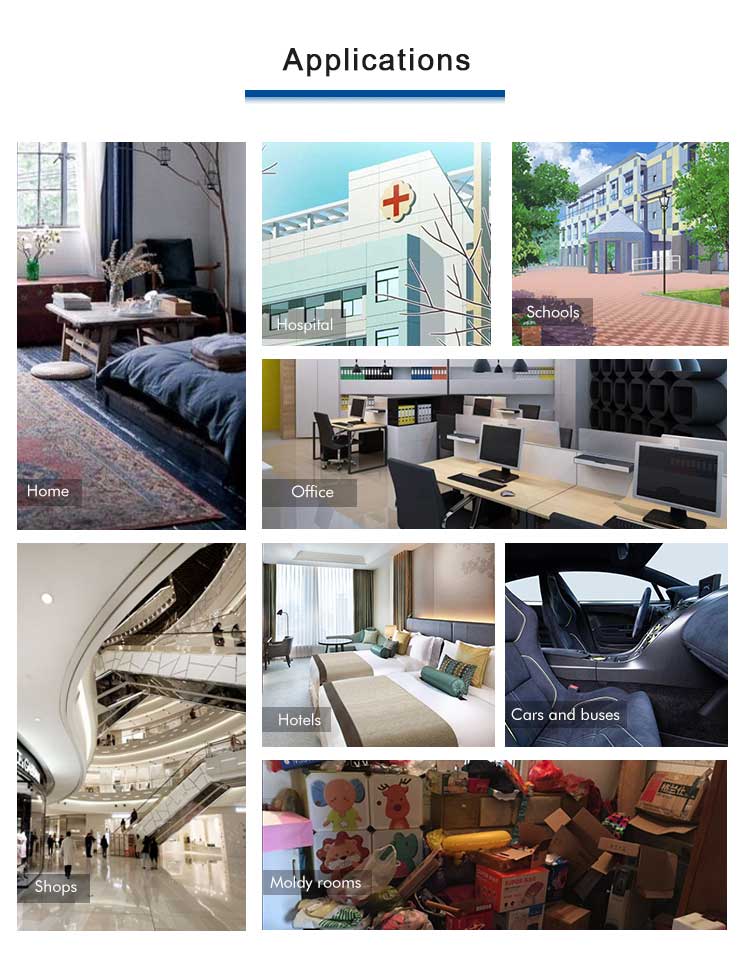The image features a header labeled "Applications" and presents a series of generic photos depicting various locations and venues. These locations include:

- **Home**: A residential setting.
- **Hospital**: A medical facility.
- **Schools**: A modern, computer-generated image of a school building.
- **Office**: A typical workplace environment.
- **Shops**: A bustling three-story mall.
- **Hotels**: An upscale, luxurious hotel.
- **Cars and Buses**: The view from the passenger seat towards the driver, showcasing the steering wheel, dashboard, and middle console.
- **Moldy Rooms**: A storage area filled with boxes in a moldy condition.

Each photo appears to be a placeholder, likely indicating that the site is still under construction and that the actual content has yet to be finalized.